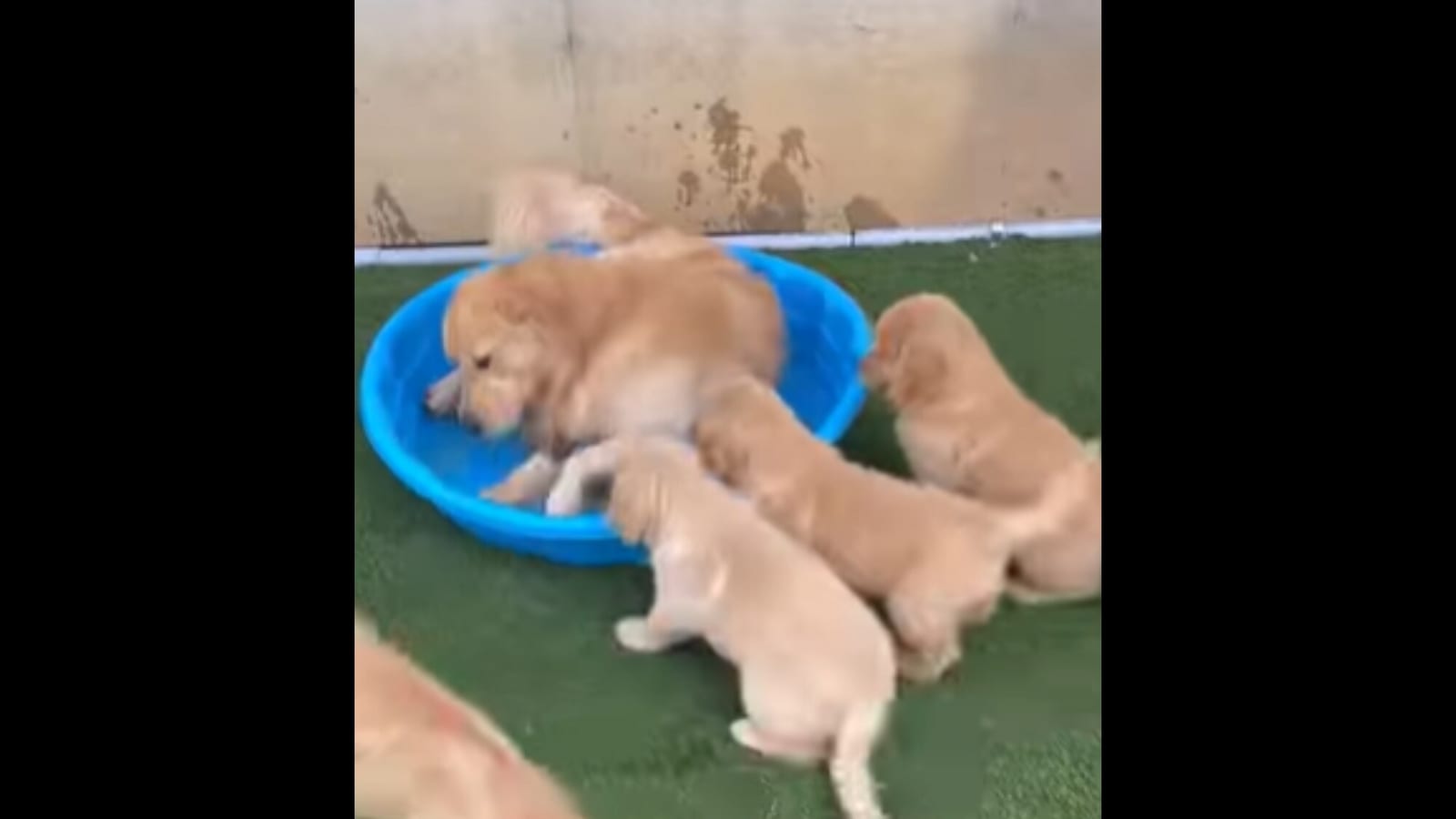In the blurry, square photograph framed with thick black bars on either side, a scene unfolds of a gold lab and three identical puppies in a small, bright blue plastic kiddie pool set on synthetic green grass. The pool, previously filled with water as indicated by the splashes on the surrounding tan-colored concrete wall, is now empty. The gold lab, probably an adult, appears to be digging in the pool, its blurred form suggesting motion. Outside the pool, three smaller, tan-colored puppies—identical to the larger dog—stand, eagerly looking towards the pool. The environment is further characterized by a white pipe running along the bottom of the wall, with darker splotches on the concrete, adding to the lively backdrop. In the lower left-hand corner, a patch of tan fur hints at the presence of another dog, slightly out of frame.